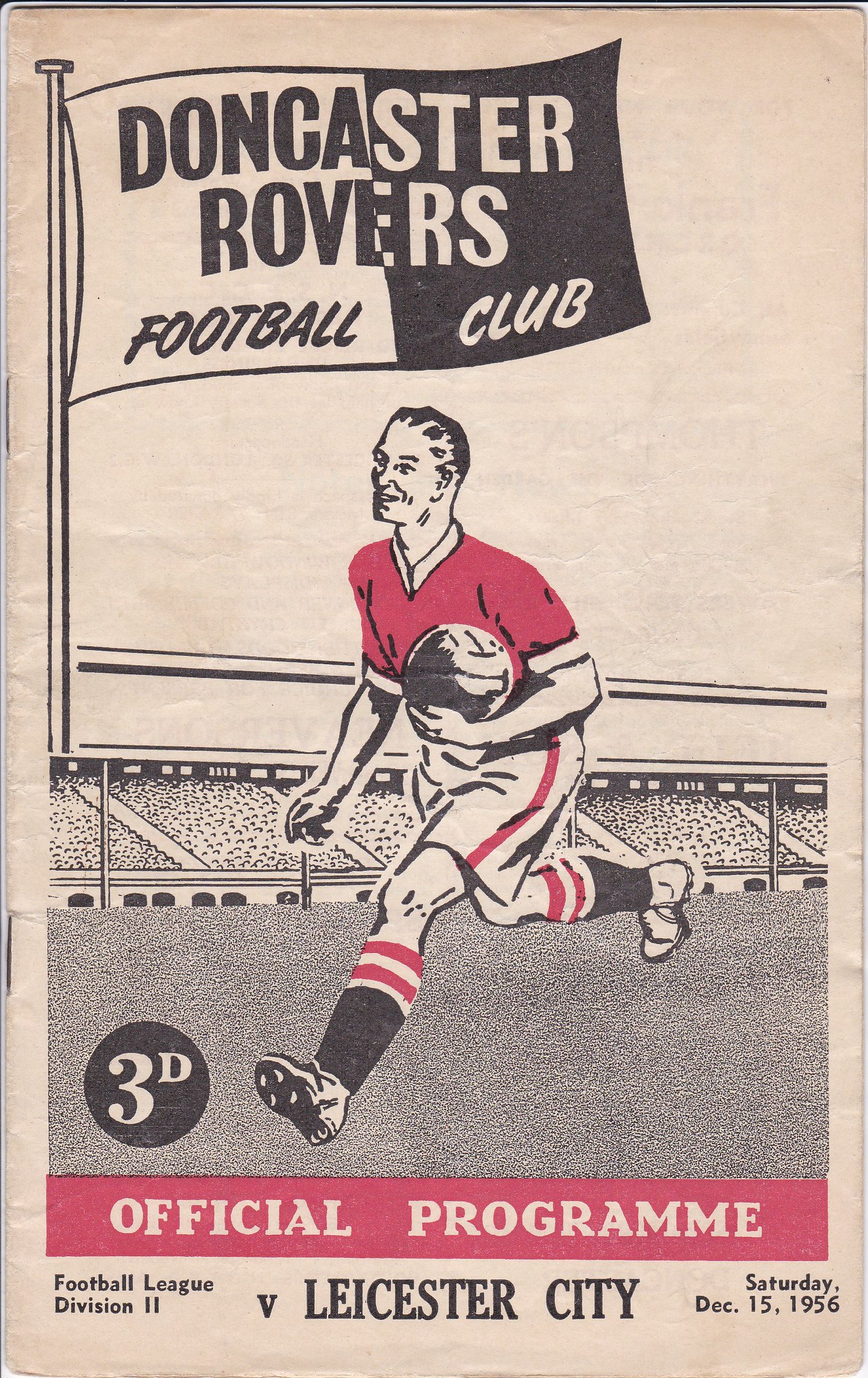The front cover of the program for the Doncaster Rovers Football Club, dated Saturday, December 15, 1956, versus Leicester City in Football League Division 2, features a central graphic drawing of a football player. The illustration, which is not photorealistic, depicts the player running across a field while carrying a football. The player's jersey is notably colored in red, with matching red accents on the shorts and socks. Above him is a large pennant styled half in white and half in black, bearing the name "Doncaster Rovers Football Club." The design uses a limited color palette of black, white, and red, with the text "Official Program" also highlighted in red at the bottom of the cover. This striking and clean design takes up almost the entirety of the cover, presenting a bold and classic look that would be expected for a matchday program from that era.